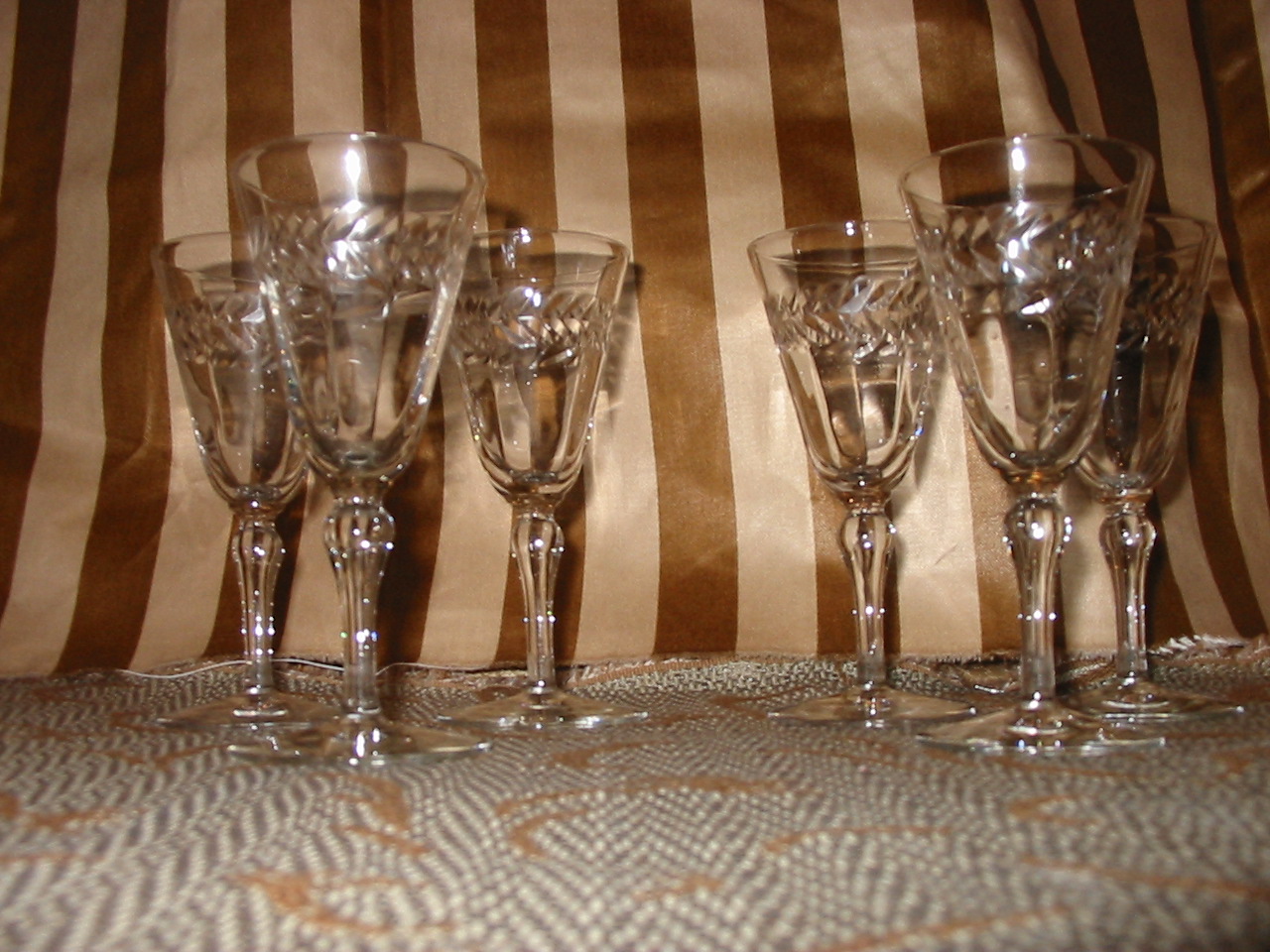A flash-illuminated photograph captures six identical wine glasses arranged symmetrically in two groups of three on a textured tablecloth. Each glass features a large, circular flat base, a slightly bulbous stem that tapers at its midpoint, and a wide, flared cup adorned with an intricate engraving of laurel-like leaves encircling the upper portion. The background showcases a smooth, satiny fabric with vertically aligned beige and chocolate-brown stripes, adding a touch of elegance and warmth to the scene. The tablecloth beneath the glasses is a blend of gray, white, and hints of yellow and orange, enhancing the overall visual contrast. The photograph tilts slightly to the right, with more space on the left, and is brightly lit, creating distinct highlights on the clear glass, enhancing the shininess of the satin fabric behind.